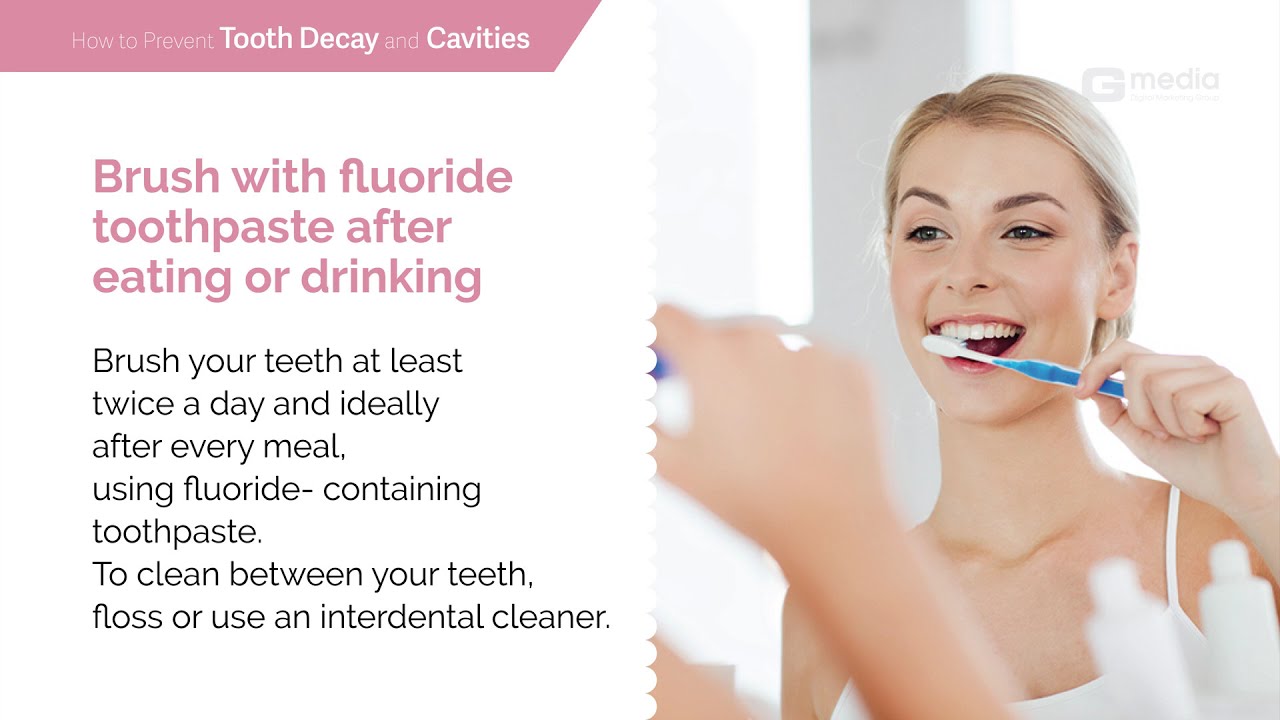The image is a detailed stock advertisement dedicated to educating viewers on how to prevent tooth decay and cavities. Set against a white background, the primary focus is on a young blonde woman, likely in her 20s, who is smiling as she brushes her teeth with a blue and white toothbrush. Her hair is tied back, and she is depicted looking into a bathroom mirror, with her reflection visible in the image. 

In the upper left corner, a prominent pink box contains the title "How to Prevent Tooth Decay and Cavities" in white letters. Below this header, additional tips are displayed in pink and black text: "Brush with fluoride toothpaste after eating or drinking," "Brush your teeth at least twice a day and ideally after every meal using fluoride-containing toothpaste," and "To clean between your teeth, floss or use an interdental cleaner."

To the right of the textual information, the girl brushing her teeth is dressed in a white tank top, fitting seamlessly into the clean, white-themed room. In the top right corner, the image also features a logo with the inscription "G-Media" and "Digital Marketing Group," suggesting the origin of the advertisement. The overall ambiance of the image conveys a clean, hygienic, and health-focused message.